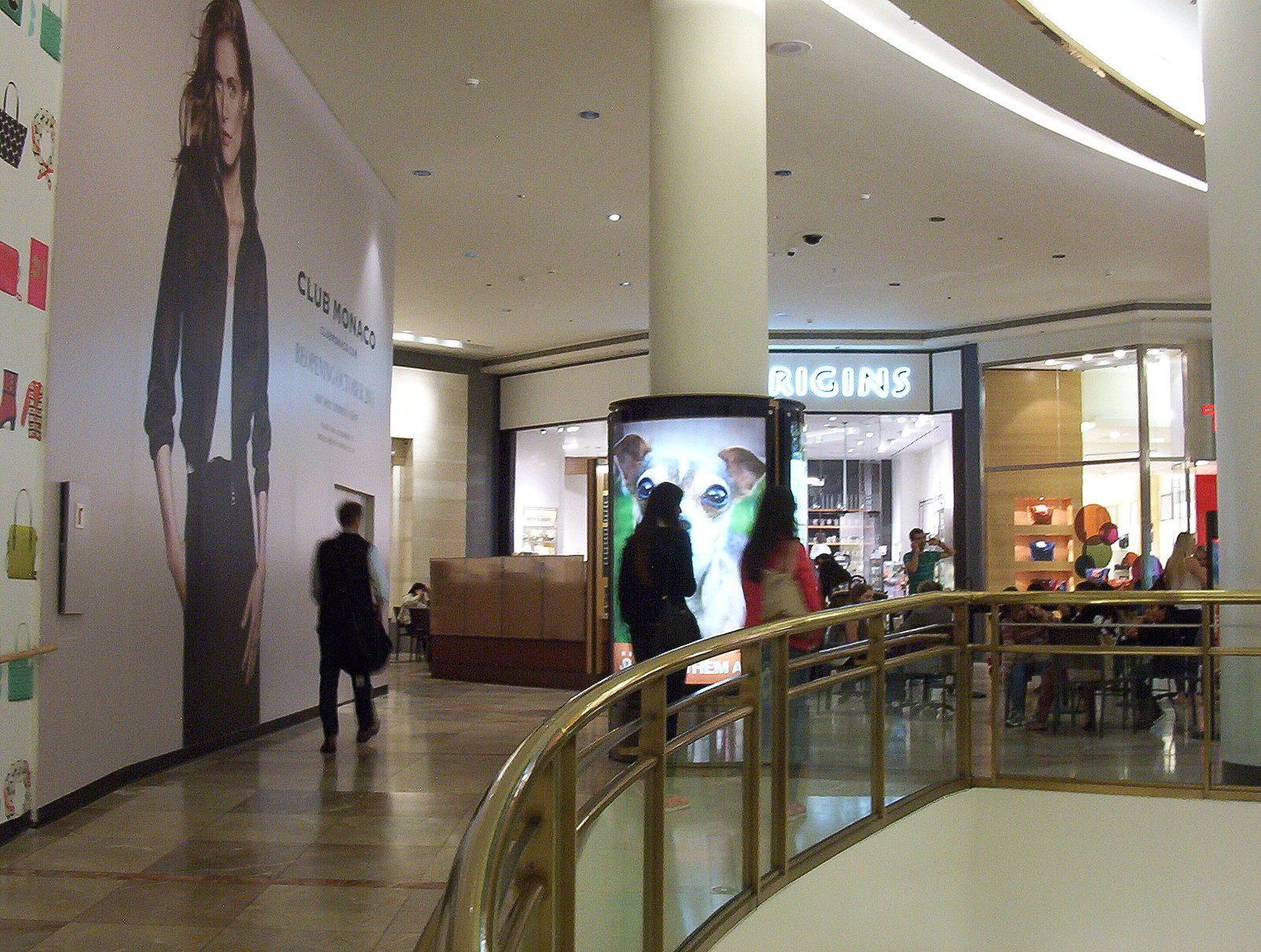This image captures the interior of a shopping mall's upper floor. Dominating the scene is a curved glass railing that runs along the edge of the open balcony, ensuring safety for mall-goers. Prominently displayed on the left-hand side is a large, stylish sign for "Club Monaco," set against what appears to be a temporary partition, suggesting that the store is under construction and preparing to open soon. Below the sign is a well-dressed model, adding an upscale touch to the advertisement. 

A large column rises in the center of the image, partly obscuring the view of two women walking nearby. This column features an ad with a photograph of a Jack Russell Terrier, adding a charming, eye-catching element to the otherwise sleek, modern setting. In the background, we see multiple storefronts, including one with an illuminated sign that says "Origins," as well as an outdoor café with seating areas. The environment suggests a bustling, yet sophisticated atmosphere, with various people walking and browsing through the mall. The overall scene is both dynamic and inviting, capturing the essence of a contemporary shopping experience.